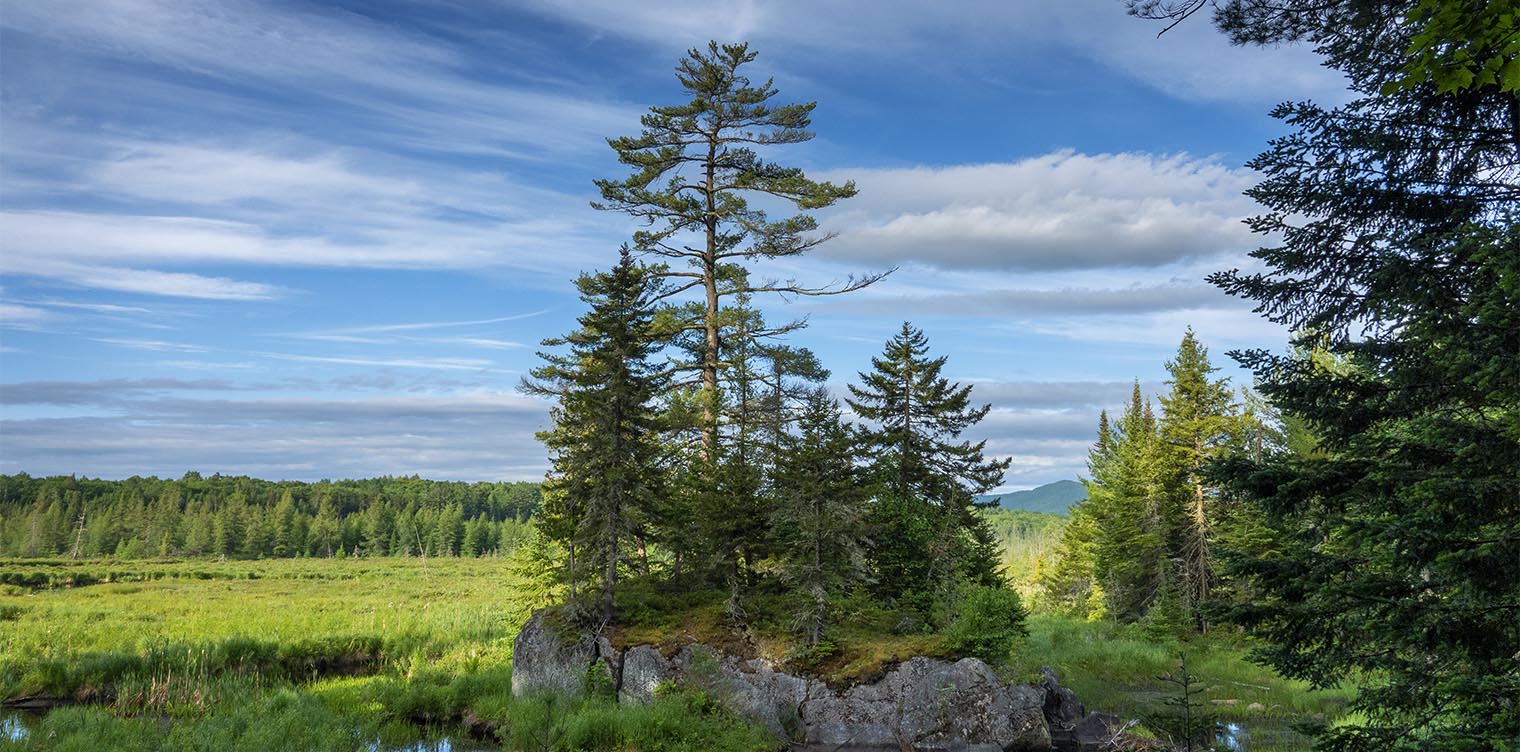This horizontal rectangular photograph captures a scenic countryside landscape. The foreground features an outcropping of gray rock with clusters of evergreen trees growing from it, flanked by more trees on either side. On the right edge, a tall tree extends out of the frame, while to the left, a medium-sized evergreen stands beside shorter ones, all atop a small, elevated mound. In front of this mound, a stream winds by, bordered by white and brown stones and patches of green vegetation.

As the scene extends into the mid-ground, a grassy field stretches out on the left, eventually giving way to a dense tree line. Beyond this in the distance, rolling hills and a mountain are visible, adding depth to the landscape. The backdrop is graced with a rich blue sky adorned with horizontal streaks of white clouds. The image, taken during the daytime, creates a serene and untouched natural panorama, emphasizing the unspoiled beauty of the wilderness.